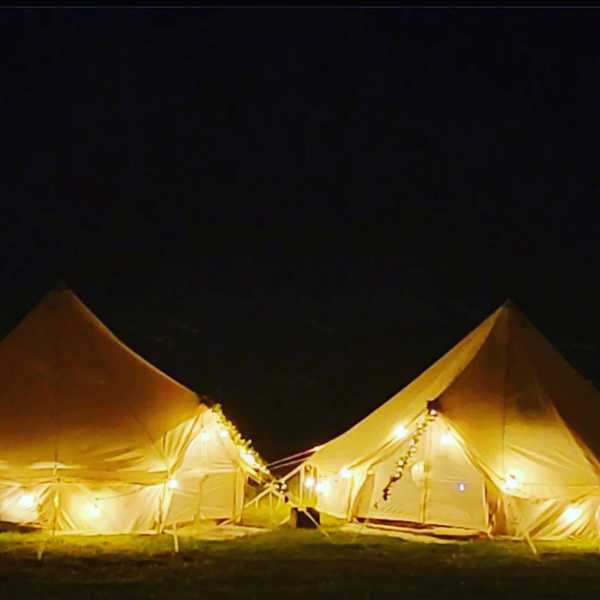The image features a vertical rectangular scene captured at night, where the top two-thirds of the frame are enveloped in darkness. In the foreground, there are two large, triangular-shaped tents side by side, each characterized by pointed tops. The tents are dark yellow with the bottom portions glowing in a lighter yellow hue due to illumination from inside. The interiors are brightly lit, casting a warm, welcoming glow. The doorways, located at the fronts of the tents, are flat and appear to have flaps for easy entry. The tents are anchored to the ground with visible cables or ropes, enhancing their triangular shape. A string of lights cascades down the front cables of each tent, further illuminating the entries and adding to the vivid ambiance. The ground beneath the tents is mostly dark, with subtle hints of dark green. This creates a stark contrast against the black sky and heightens the focus on the vividly lit tents.